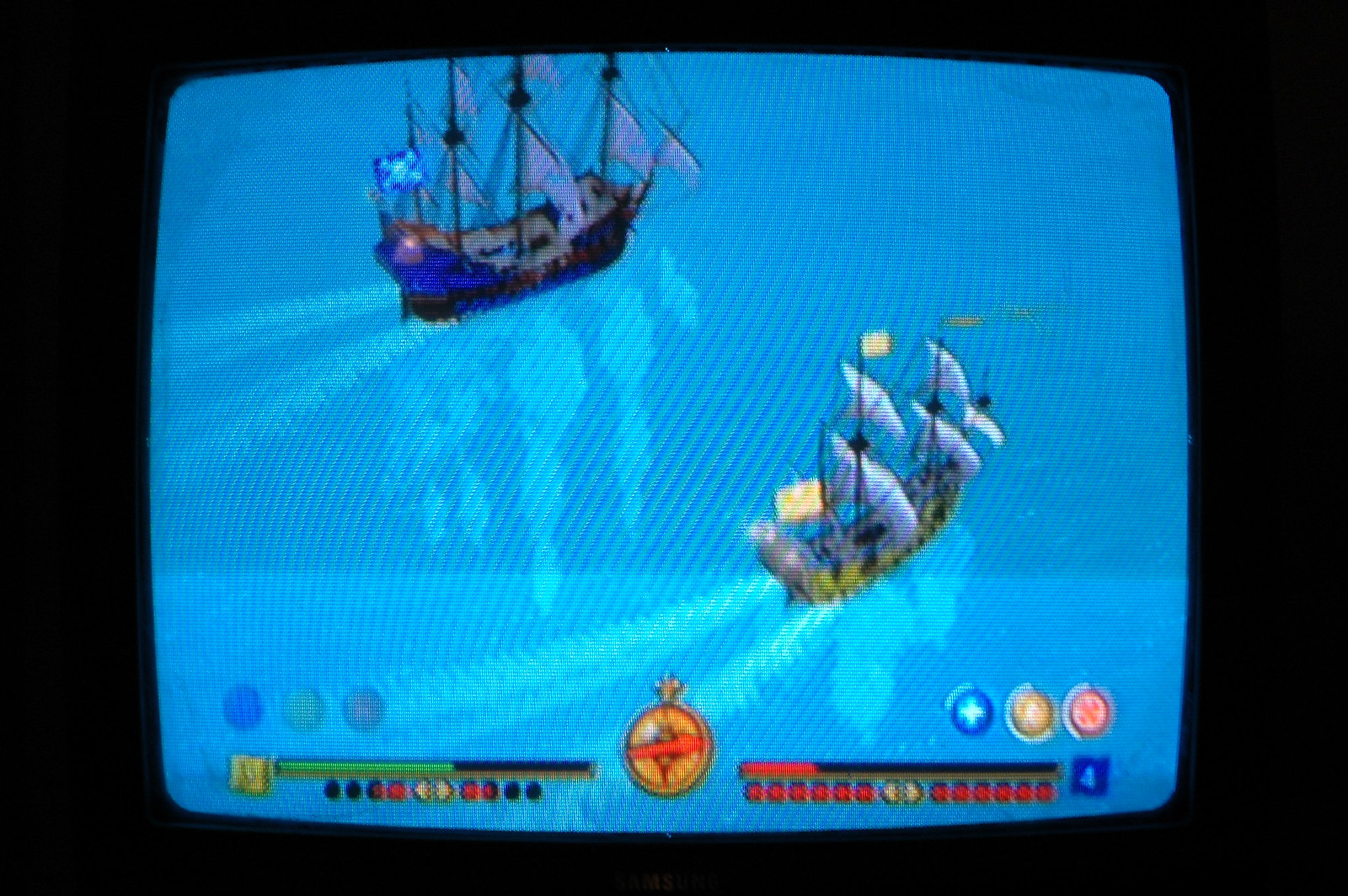This is a vibrant color photograph, evidently a screenshot from a video game. Dominating the entire screen is a picturesque expanse of water, showcasing a blend of beautiful blue hues, ranging from turquoise to aqua. The water, simply illustrated and far from photorealistic, sets the scene for two classic sailing ships from the 17th to 19th centuries, complete with large, billowing white sails. One ship is positioned in the upper left-hand corner, while the second ship is located towards the lower right-hand corner of the image. At the very bottom center, a yellowish disc-shaped icon featuring a grey oblong design is visible. Additionally, a series of colored dots are displayed at the bottom of the image, consisting of red, blue, and yellow hues, adding further detail to the game's interface.